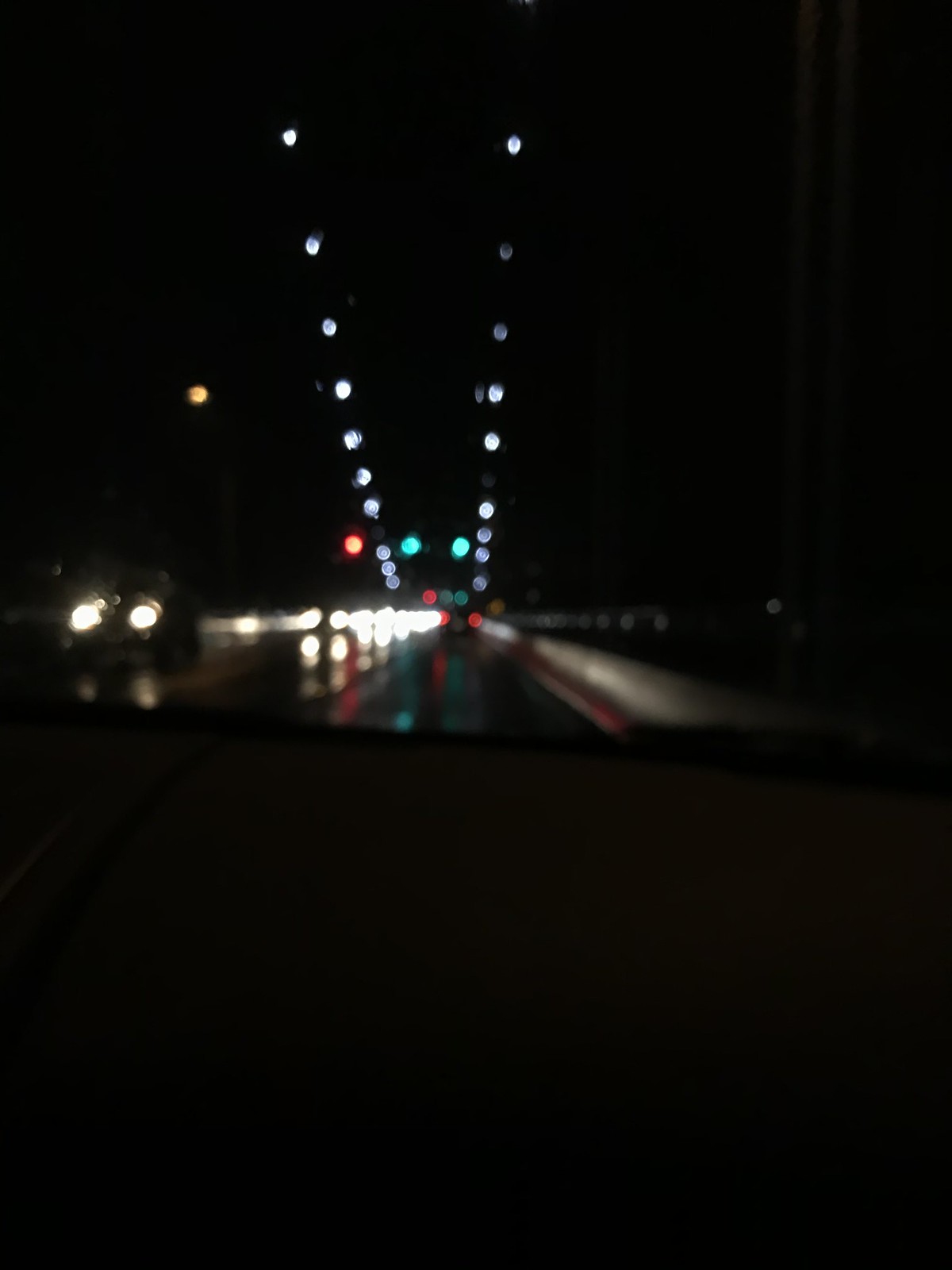In this image, the overall scene is quite dark and the quality is notably poor. The photo is blurry and has a low resolution, making it difficult to discern finer details. Despite the fuzziness, it appears to depict a road with cars traveling in opposite directions on either side. Streetlights above the road emit a mix of brown, white, and blue hues, which dimly illuminate the area. On the left side of the image, one car is particularly noticeable because its circular front headlights are turned on, casting a white light. The lower portion of the image is largely obscured in black, adding to the overall indistinctness of the scene.